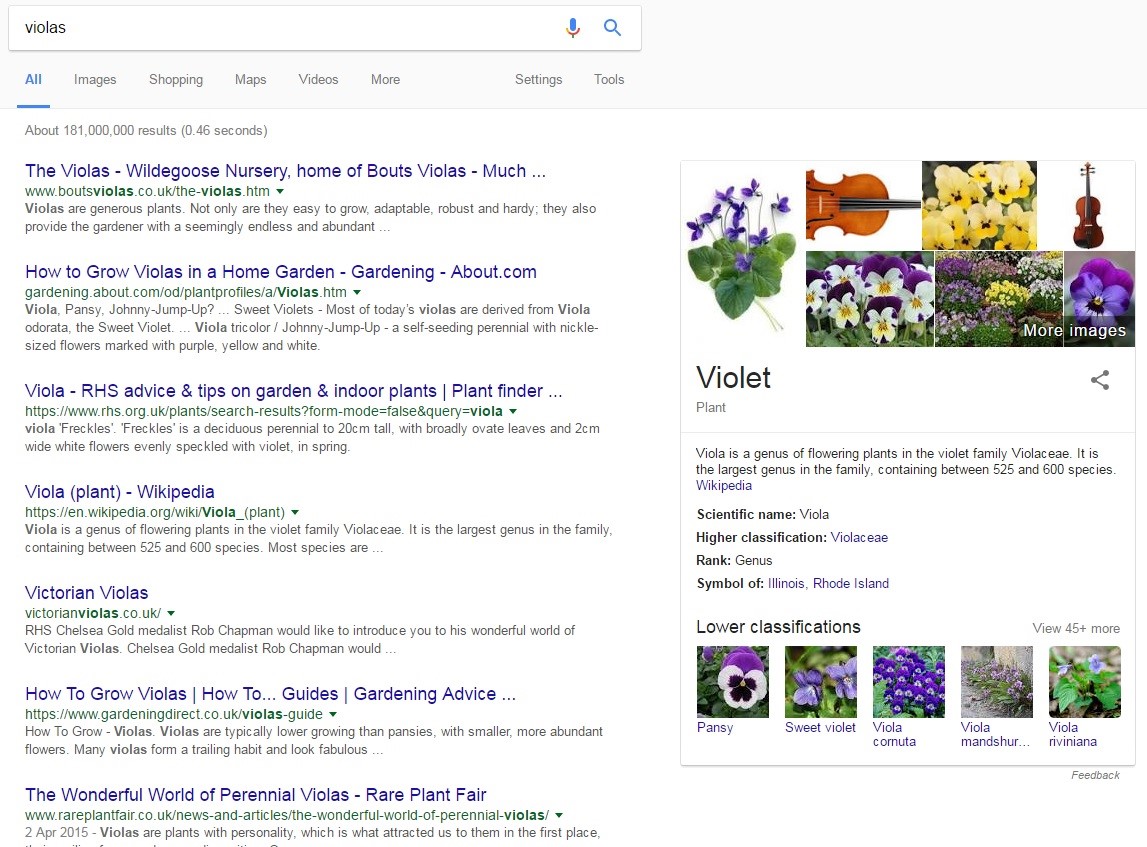The image showcases a Google search results page following a query for the term "Violas." At the top, the "All" results category is selected, indicating that the page displays all types of search results. On the right side, a knowledge panel is visible, beginning with the word "Violet" and followed by the term "Plant" in gray. The panel provides a brief description, stating that "Viola is a genus of flowering plants in the Violet family." It further elaborates that Viola is the largest genus in the family, comprising between 525 and 600 species, according to a source from Wikipedia. 

Additional details given include the scientific name "Viola," its higher classification, and its symbolic significance to the states of Illinois and Rhode Island. Below this information, there are smaller images representing various flowers that belong to lower classifications within the genus. 

Above the term "Violet," several images of violets are displayed, interspersed with a few images of violins, which contributes an interesting mix. 

On the left side of the page, there is a vertical list of webpage links, characterized by bright blue titles and accompanied by brief excerpts of gray text underneath each link, summarizing the content of the respective pages.

Overall, the detailed layout provides comprehensive information about Violas, blending visual elements with textual descriptions to enhance the search experience.